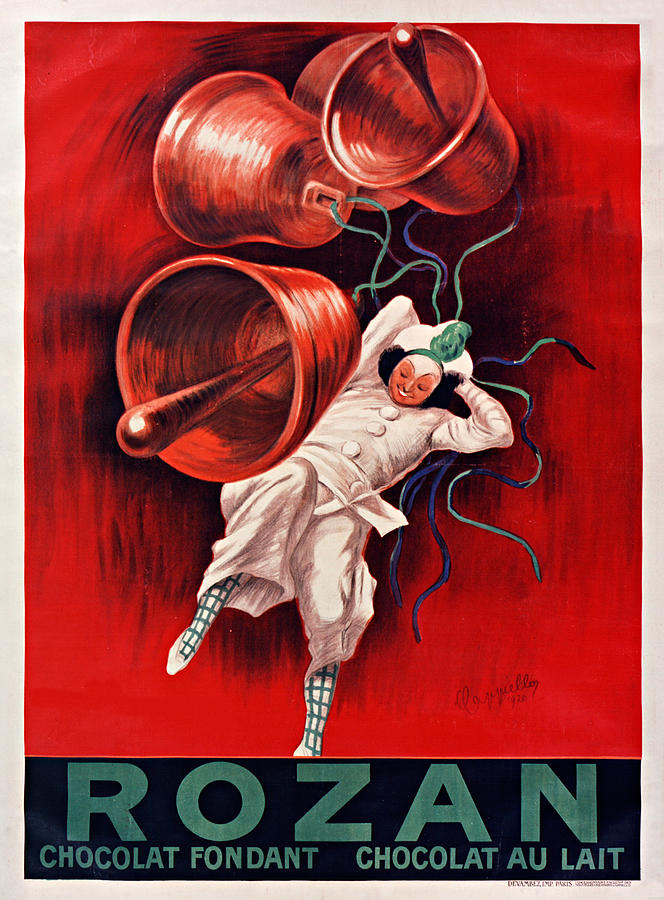The image is a vibrant, color illustration rendered in a posterized wall art style, predominantly featuring shades of red with a striking central figure. The background showcases bold red paintbrush strokes creating a dynamic atmosphere accented by a black horizontal bar at the bottom. The central figure, potentially a woman or a man, is dressed in an all-white two-piece suit adorned with three prominent buttons running vertically down the front and a wide belt. The figure is smiling, their short dark hair peeking out from beneath a distinctive triangular-shaped white hat, which features a teal feather plume and teal accents.

Above the figure, three copper-colored bells are depicted mid-ring, each attached to blue, teal, and green ribbons that seem to cascade from the figure's hat. The bells are intricately detailed, with visible clappers inside, oriented in various directions to create a sense of motion. The figure’s socks are a blue and white checkered pattern, extending into white shoes, adding to the overall grid-like design.

Below the figure, the black bar contains aqua-colored text that reads "Rosanne, R-O-Z-A-N," and beneath it, in smaller aqua text, "Chocolate Fondant." To the right, it says "Chocolat Aulat, L-A-I-T," describing likely chocolate products.

The entire artwork is framed by a white border, and there is a signature in the red area that appears illegible. Overall, the vivid color scheme and dynamic elements of this advertisement convey a sense of lively celebration and artisanal charm.